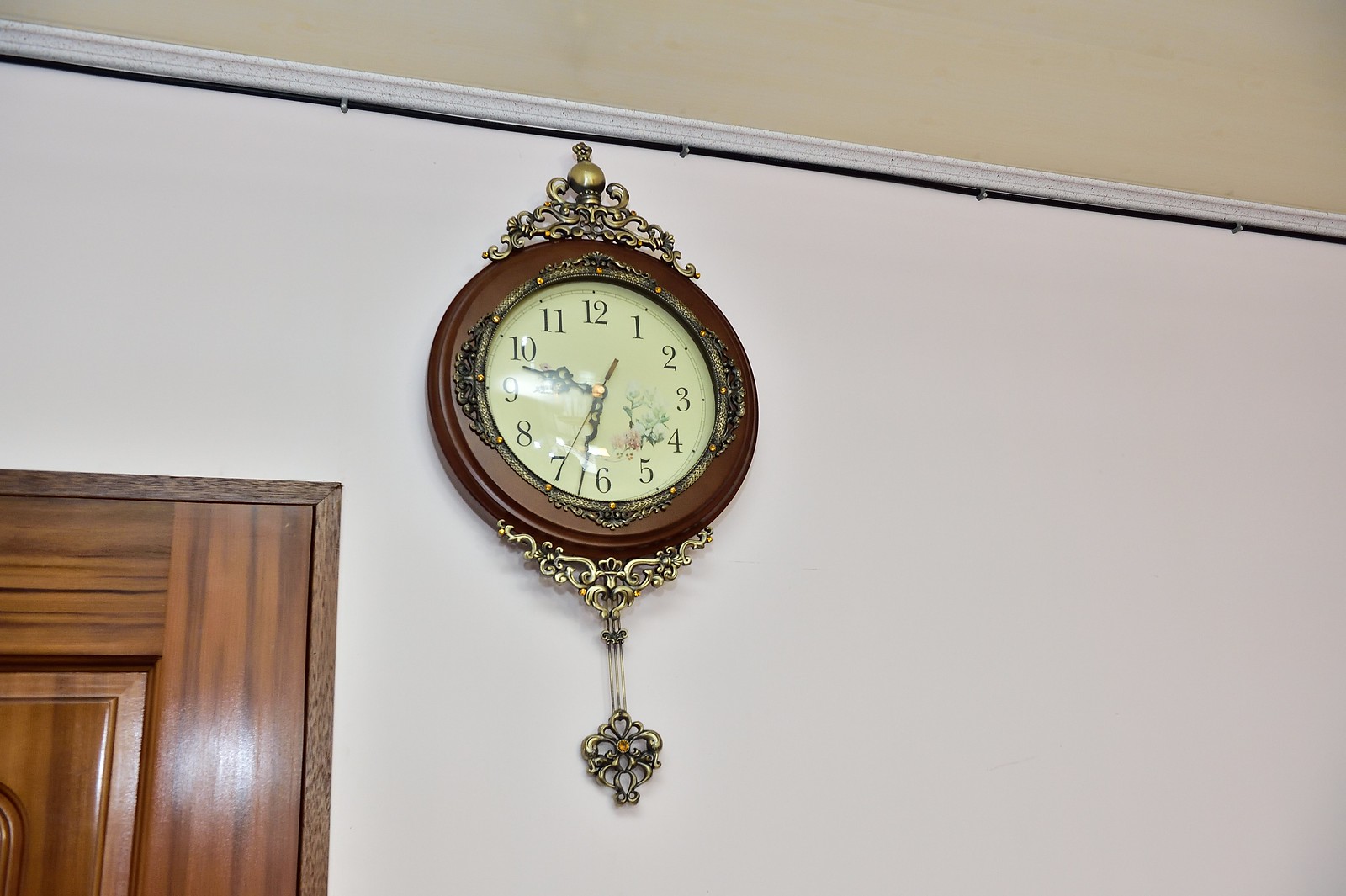The image features a vintage clock prominently displayed on an off-white wall, blending subtly with the creamy beige ceiling above. Above the clock, a black coaxial cable is secured with u-shaped tacks, trailing along a section of white crown molding. The lower left side of the image reveals the upper part of a varnished wooden door and its matching frame.

The clock has a light tan, yellowish face adorned with a delicate floral pattern located between the three and five positions, featuring flowers in shades of blue, pink, and red, with greenish stems. The outer border of the clock face is encased in dark varnished wood, and intricate metal decorations embellish the top, bottom, and sides of the clock.

The clock hands, including an ornate hour hand and a dark gold minute hand, are designed with elaborate, irregular curves. Below the clock face hangs a decorative pendulum-like feature that may swing back and forth, contributing to the clock’s classic, old-fashioned charm. The clock indicates the time as approximately 9:33 and 35 seconds.